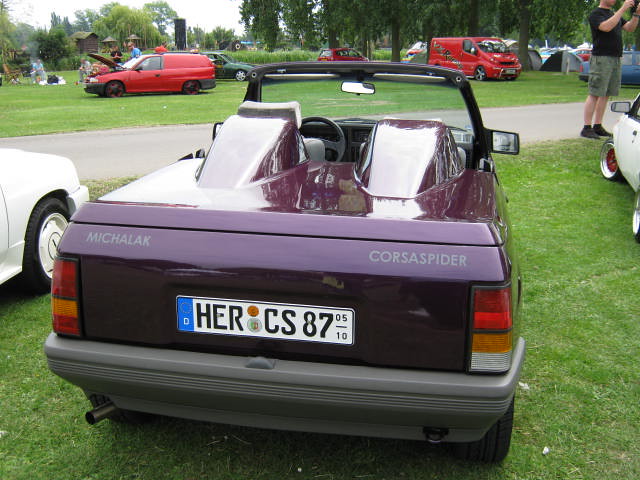The image captures a lively car show or gathering set in a park-like area with well-mowed green grass. Dominating the foreground is a maroon Mecalac Corsa Spyder, a European convertible with the roof down, distinguished by its long white European license plate with a blue panel on the left side. The Spyder is parked diagonally on the grass between two white cars, whose exact models aren't clear. Surrounding it are various other vehicles, including multiple red vans, with one displaying an open hood, possibly indicating a mechanical issue. The background reveals a road cutting through the scene, with more cars parked on the opposite grassy side. Among these, a large red Jeep stands out. There are also several tents visible behind some trees, with people engaged in activities like cooking around a small campfire. The atmosphere suggests a communal event for car enthusiasts, further emphasized by numerous attendees, including a Caucasian man near a white vehicle, presumably taking photos or videos.